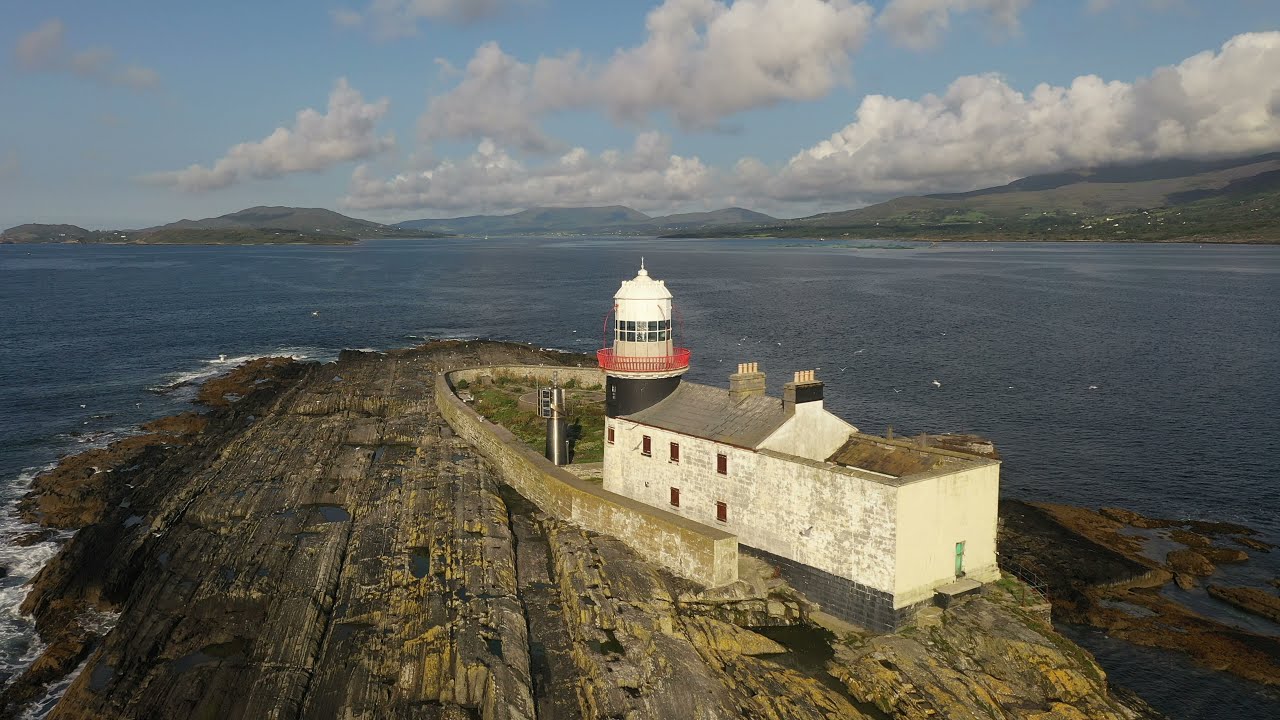This photograph captures a stark lighthouse perched on a rugged rock outcropping jutting into tranquil waters. The lighthouse itself is a striking color block of bright white on top and deep black at the base, adorned with a vivid red metal railing circling its upper section. A rectangular building adjacent to the lighthouse, reminiscent of an Alcatraz-type structure, features six shuttered windows with brick-red shutters. A large steel cylinder emerges from the ground to the left of the structure. The rocky outcropping, devoid of vegetation and hued with a yellowish tint, contrasts sharply with the smooth water that surrounds it on three sides. Waves gently lap against the shore on the left, while the right side remains calm. In the distance, a backdrop of hills and mountains stretches across the horizon under a mostly blue sky dotted with fluffy white clouds, enhancing the serene yet dramatic landscape.